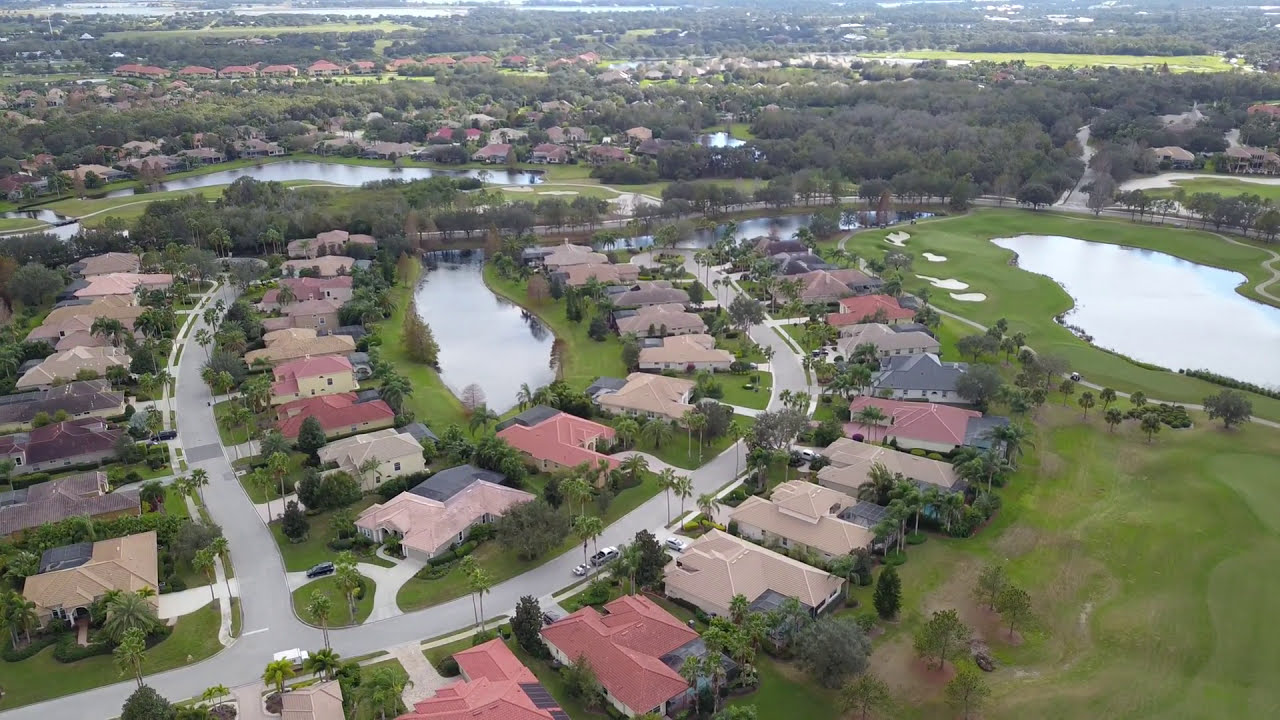An aerial photograph captures a sprawling suburban residential area characterized by rows of single-family homes arranged in semi-circles. The majority of these homes feature distinct red roofs, with some sporting cream, gray, or even blue hues. Intersecting the homes are gray roadways set among lush, green, grassy areas that give the appearance of manicured lawns or possibly a golf course. Dotted throughout the scene are several vivid blue ponds, with a prominent one in the center left and another larger pond to the right, and additional smaller ponds visible in the distance. The entire area is peppered with numerous trees, particularly dense in the upper right of the photograph, contributing to an overall verdant and tranquil atmosphere. The scene extends seamlessly from the foreground to the horizon, emphasizing the expanse of the development and the natural elements that intermingle with the residential units. The photograph, taken from approximately 100 feet above, offers a detailed and vibrant view of this suburban neighborhood on a clear day with a reflective light blue sky.